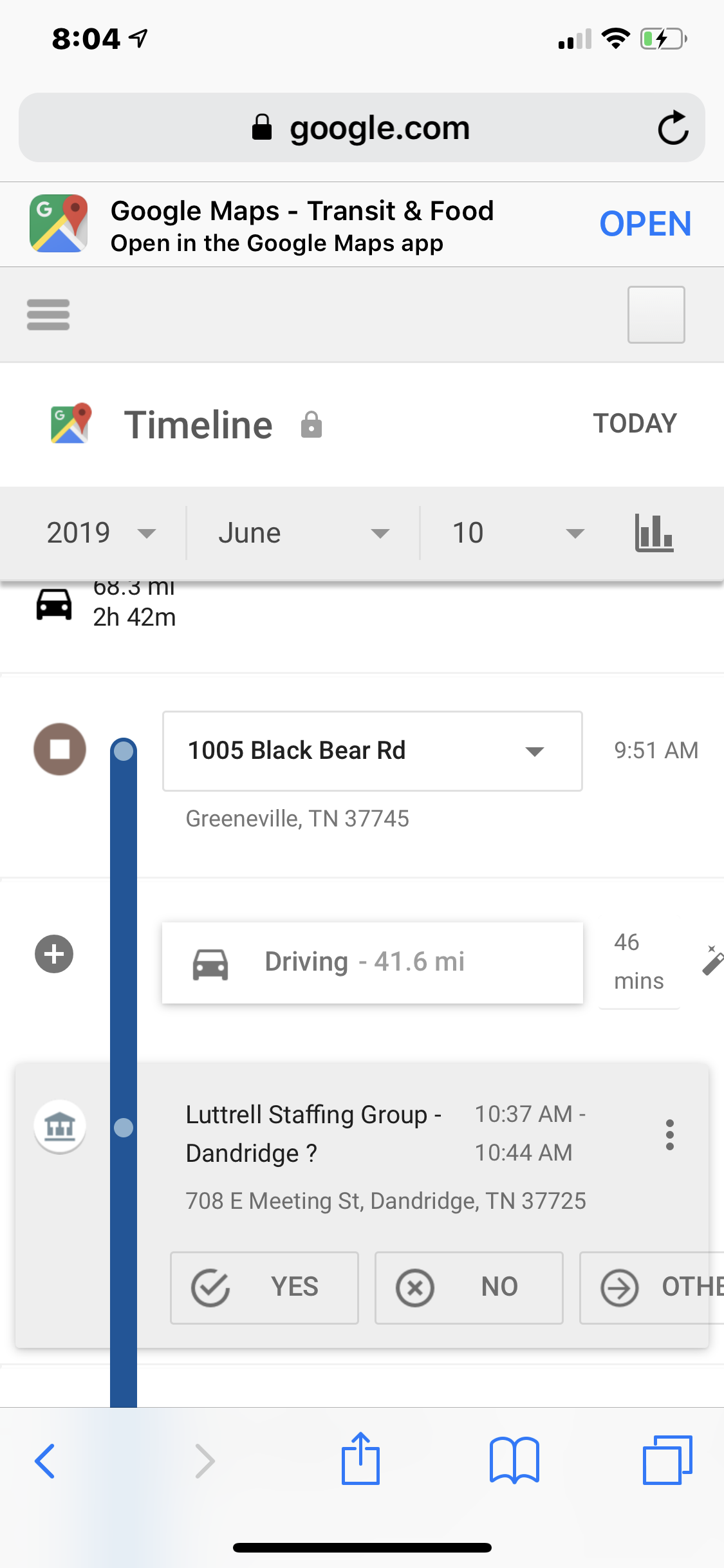This screenshot from a phone displays several interface elements and notifications:

At the top of the screen, the time is displayed as 8:04 AM, with a weak signal indicator and a nearly depleted battery icon. Below, there is a gray box featuring a locked padlock icon indicating secure content, followed by the text "google.com" and a refresh button.

Underneath this, the screen shows Google Maps sections: "Transit" and "Food" categories alongside "Open" indicators, with "Maps" specifically highlighted in blue as the currently selected option. An adjacent locked icon appears next to "Timeline" with data entries listing today’s date, June 1st and June 10th, 2019, and a bar graph on the right.

Further down, another teal progress line is directed from "1005 Black Bear Road, 9:51 AM, Greenville, Tennessee" showing a driving distance of 41.6 miles taking approximately 46 minutes to reach "Luttrell Staffing Group, 708 East Meeting Street, Dandridge, Tennessee." Here, the "Yes" option is checked.

At the very bottom, navigation buttons including back, forward, and a close button are presented. Additionally, there is an icon representing multiple overlapping pages, suggesting the presence of other open tabs or windows.